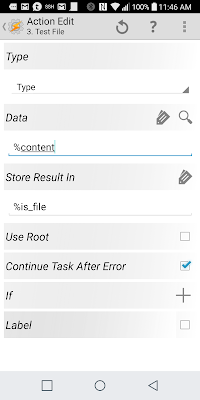The screenshot displays an interface from an application on a mobile device. The background is primarily a grayscale theme, where sections alternate between gray and white. At the top of the screenshot, there are standard system icons such as Gmail, battery status, and Wi-Fi signal, indicating that it is a mobile device.

Beneath the system icons, a gray text box labeled "Action Edit" is positioned to the left, accompanied by a few icons, including a back button and a question mark. The interface consists of multiple sections, each with a gray header and a white content area. The first section includes a gray box titled "Type" and a white drop-down menu also labeled "Type."

This pattern continues with other sections such as "Data," "Content," "Store Result" (in a gray box), followed by white drop-down menus for each category. Additional options like "File," "Use Root," "Continue Task After Error," "If," and "Label" are listed under different categories. At the bottom of the interface, there are several buttons, including "Back" and "Done."

The organized layout and functional icons suggest this is part of a settings or options menu within the app, providing various customizable features and inputs for the user.